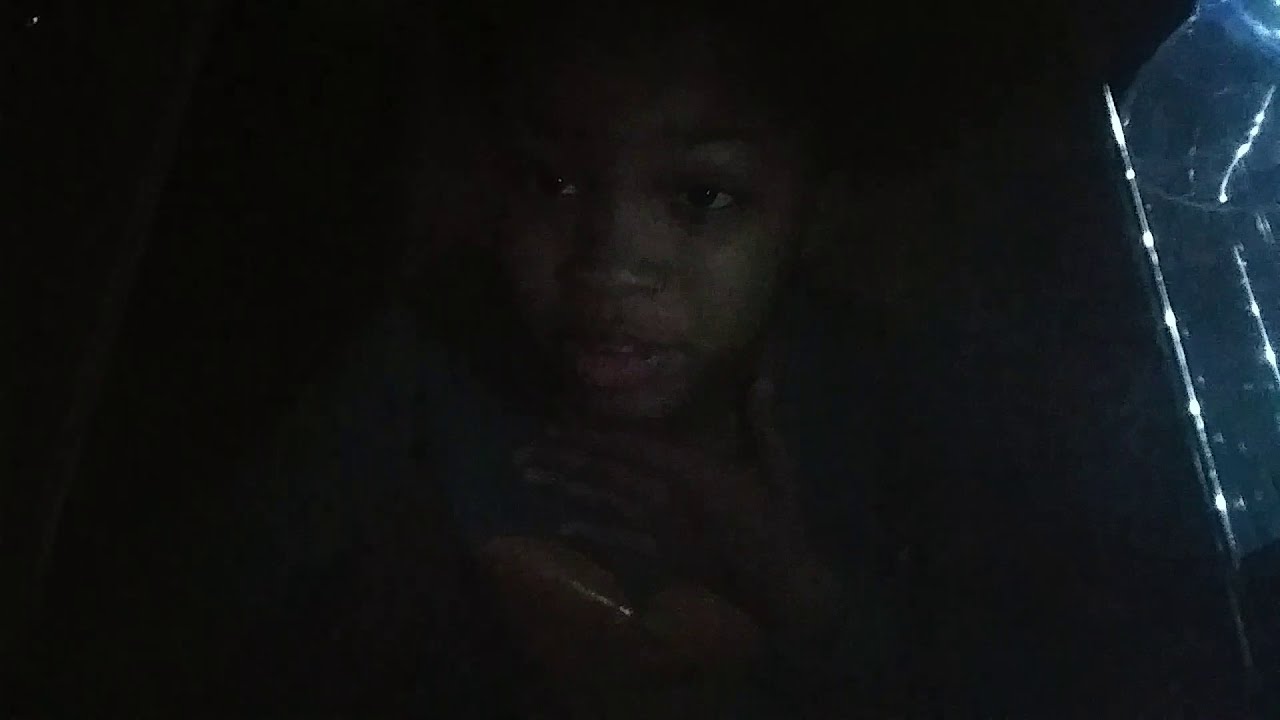This photograph deeply shrouded in darkness features an African-American child with dark skin, sitting and gazing upward toward the top right. The child's wide-open eyes and slightly parted, plump lips are softly illuminated by a faint light visible on the right side of the image. The child is wearing a t-shirt with a discernible but indistinct design, possibly a yellow heart. Their left hand lies flat against their chest, suggesting a gesture of comfort or contemplation. The surrounding environment is pitch black, making it difficult to discern fine details or the exact setting. However, a blue, transparent, and partially curved plastic tube can be seen to the right, while a wooden pole or bar might be present on the left, adding to the mysterious aura. The source of the light appears to be natural, perhaps moonlight filtering through a scratched or weathered window, suggesting the child might be seated in a parked vehicle or a similarly enclosed space.